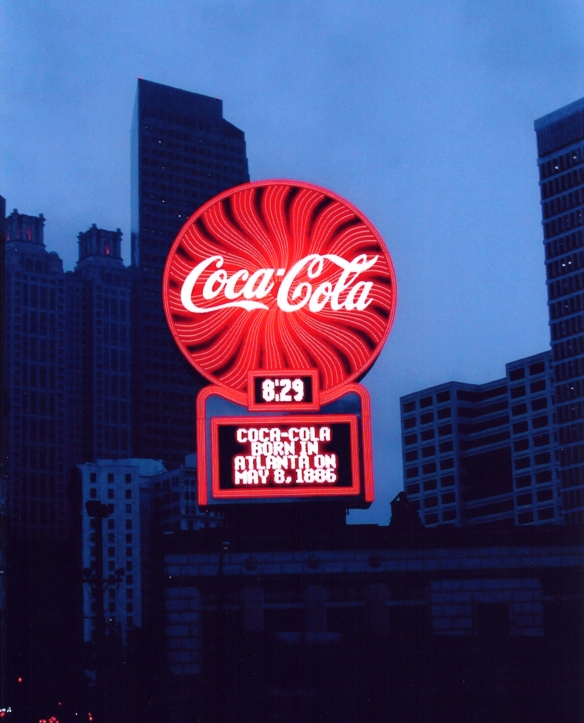In this photograph, a vibrant red circular Coca-Cola marquee stands out against a backdrop of darkly colored buildings and skyscrapers under a gray, evening sky. The sign features a red and black wavy pattern with the iconic Coca-Cola logo in white print. Below the circle, a smaller illuminated panel displays the time as 8:29 and beneath that, a marquee in a red box with a black background reads "Coca-Cola, born in Atlanta on May 8, 1886." The bottom of the image is dimly lit, revealing a street view with indistinct car lights and shadowy outlines of surrounding structures.